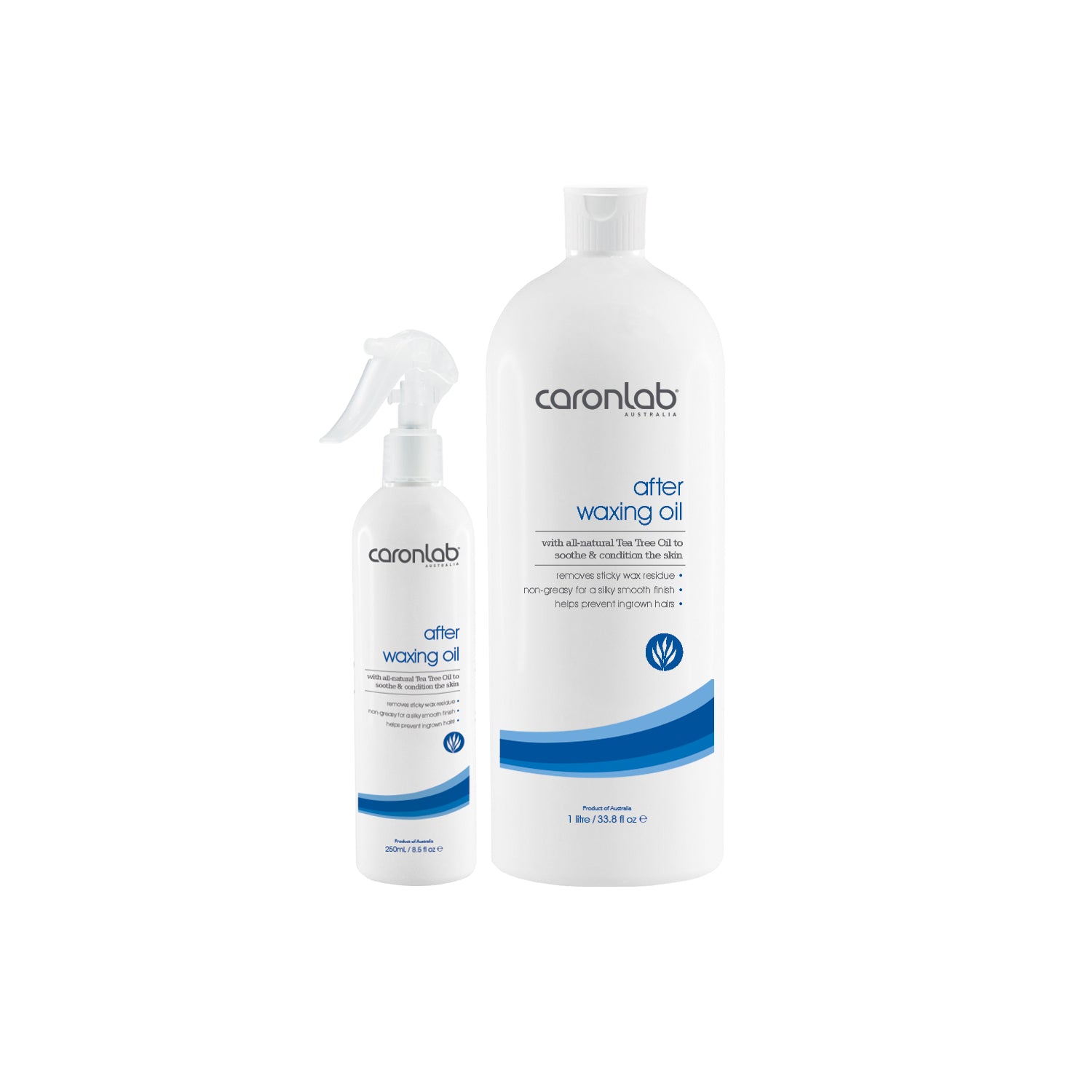This vertical image features two white containers of waxing gel from Carowind Lab. The background is plain white with no visible borders. Both containers share an identical design, characterized by blue accents and black text. The larger bottle, positioned on the right, is a one-liter (33.8 fluid ounces) container with a flip cap, while the smaller bottle on the left is a 250-milliliter (8.5 fluid ounces) spray bottle with a white pump top.

Each bottle prominently displays "Carowind Lab" at the top. Below that, in blue text, it says "After Waxing Oil." Both bottles feature three bullet points in black text that list the benefits: "Removes sticky wax residue," "Non-greasy for a silky smooth finish," and "Helps prevent ingrown hairs." Additionally, the labels mention that the product contains all-natural tea tree oil to soothe and condition the skin. A logo with a blue circle and white leaves appears beneath the text.

Five horizontal bands of different shades of blue adorn the lower portion of each container. At the very bottom, the smaller bottle indicates it is a product of Australia and includes volume measurements, while the larger bottle repeats similar information.